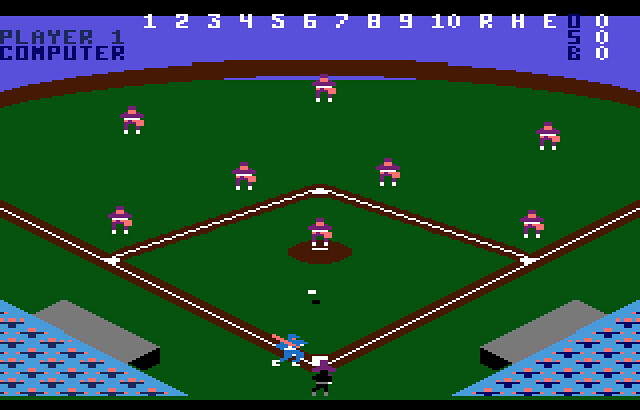This screenshot captures a moment from a nostalgia-inducing, vintage baseball video game, reminiscent of early Atari-era graphics with its simplistic, pixelated design. The scene is set in a stylized baseball stadium where a blue-shirted batter holds a stick bat, ready to swing. Behind him, a catcher clad in maroon gear crouches in position, with a black-uniformed umpire standing directly behind, overseeing the play.

The stadium is minimally detailed, with stick-figure diagrams flanking each side, representing other players and game details. The infield and outfield are populated by the "Cranberry Marine" team, identifiable by their pixelated uniforms. The scoreboard at the top of the screen displays "Player 1" against the computer opponent, alongside notations for innings and various game stats such as R, H, E, U, S, and B, all currently showing 0.

The field itself is shaded a dark green, while the background sky is an unusual violet hue, enhancing the retro aesthetic. The graphics are rudimentary and bitmap-like, characteristic of early video games, evoking a sense of simplicity and charm from a bygone era of gaming.